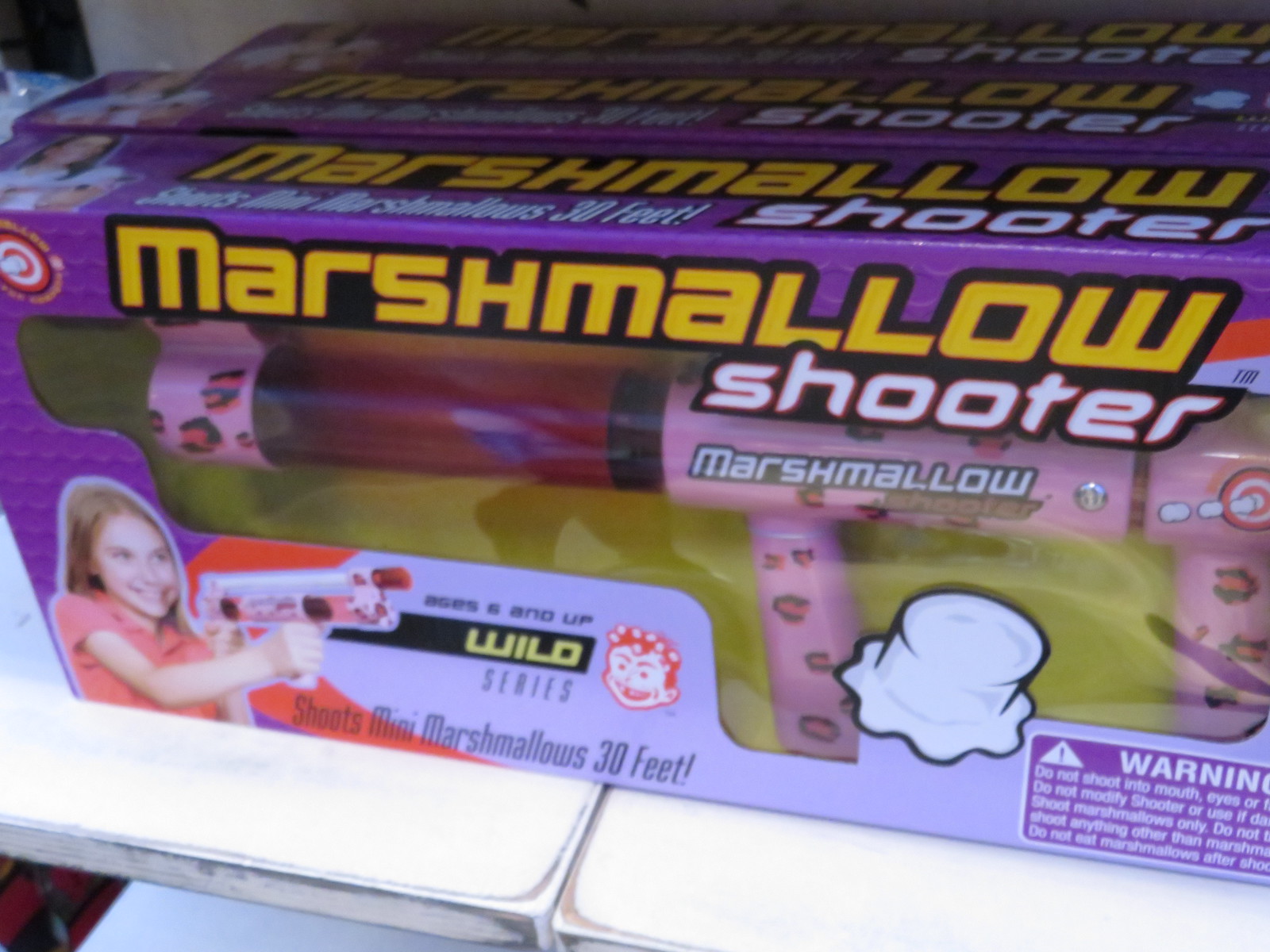This is a full-color photograph showcasing a children's toy called the Marshmallow Shooter. The packaging is primarily dark purple at the top, transitioning to a lighter lilac shade towards the bottom right. The box features the word "Marshmallow" in gold, "Shooter" in white, and prominently highlights that the toy is part of the Wild series and suitable for ages 6 and up. The toy itself resembles an old-fashioned pump-action gun, predominantly pink with red accents and intricate designs that are somewhat indistinguishable due to the image quality. 

A depiction on the box shows marshmallows being shot at a bullseye target, emphasizing that the toy can shoot mini marshmallows up to 30 feet. In the lower left-hand corner of the package, there is a picture of a young girl with long brown hair, wearing a reddish shirt and sporting a big smile, demonstrating the use of the toy. There are additional packaging details, including a partially visible warning label stating "do not shoot into mouth, eyes," and "do not modify shooter or use if," which repeats on multiple boxes arranged three deep on a white shelf.